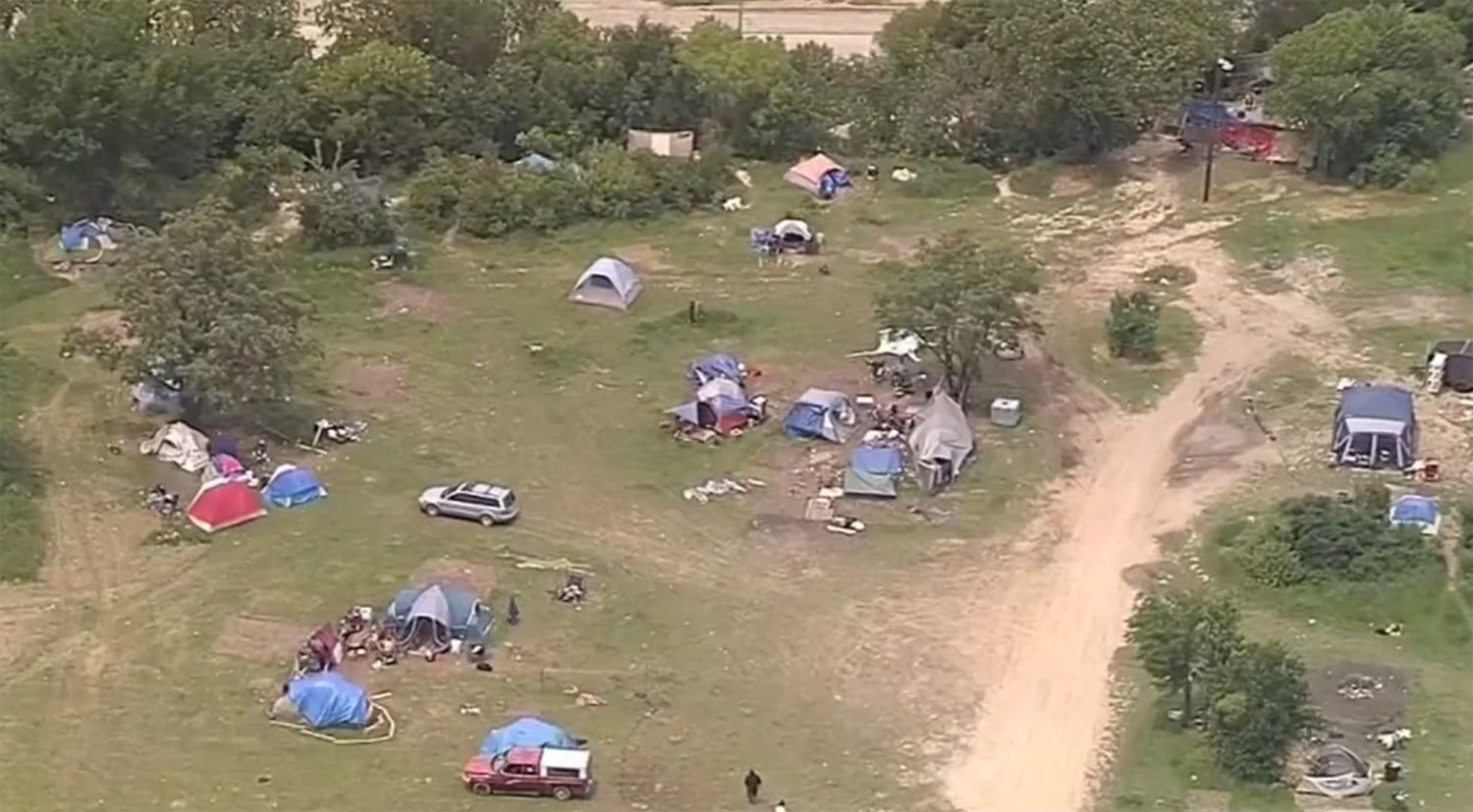An aerial, drone-captured view reveals a sprawling, loosely organized campsite that could be interpreted as either a conventional camping ground or a homeless encampment. The area, approximately the size of a football field, features a mixed backdrop of sparse trees and patches of worn grass, indicative of heavy foot and vehicle traffic. A dirt road forms a trail on the right side, providing access for cars, including a pickup truck and an SUV seen parked among the tents. Scattered across the terrain, roughly 20 tents populate the area without any apparent order, suggesting informal or long-term residency by multiple families or individuals. The overall scene exudes a makeshift, rural atmosphere, underscored by the ad-hoc arrangement of tents and the modest tree cover offering intermittent shade.